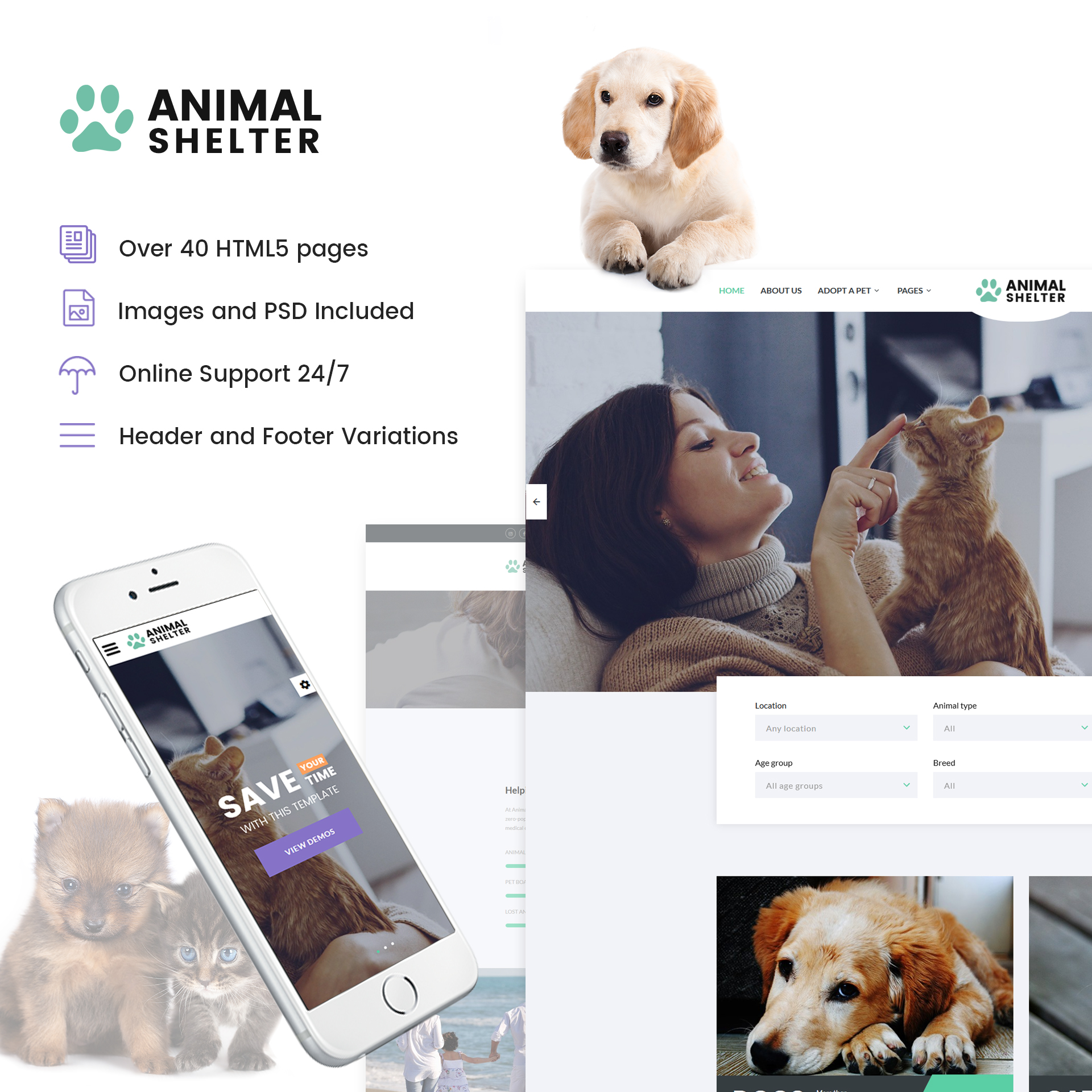This screenshot captures the homepage template of an animal shelter website, featuring a prominently displayed green paw print logo followed by the words "ANIMAL" and "SHELTER" in black, located at the top left. To the right, there's an endearing picture of a golden Labrador or Retriever puppy laying down with its paws forward and ears flopped down, looking to the left.

On the left side, beneath the aforementioned logo, there are four purple icons accompanied by descriptive text in black:
1. A stack of pages icon with the text "Over 40 HTML5 Pages."
2. An icon of an image with a folded corner labeled "Images in PSD Included."
3. An umbrella icon with the text "Online Support 24/7."
4. Three horizontal lines representing "Header and Footer Variations."

To the right of the puppy is a preview of the completed website. At the top left of this inner screenshot, the navigation menu is listed in green and black all-caps text: "HOME," "ABOUT US," "ADOPT A PET" (with a gray arrow next to it), and "PAGES" (with a gray arrow next to it). The same animal shelter logo is repeated at the top right.

Below this navigation menu, there’s a large horizontal image of a smiling woman with lighter skin and dark hair, wearing a grayish turtleneck sweater. She is gently touching the nose of an orange-and-white kitten with her hand, which has a silver or white gold ring on the ring finger. The background reveals a white desk, a black wall, and possibly a computer screen.

Below this image, there are dropdown menus styled within text boxes:
- Location (default is "Any Location" in gray)
- Age Group (default is "All Age Groups" in gray)
- Animal Type (default is "All" in gray)
- Breed (default is "All" in gray)

Further down are horizontal images of animals, including an adult golden Labrador or Retriever lying down with reddish ears, looking at the camera with dark eyes.

On the left side of this web page preview, there’s an image of a phone displaying the mobile version of the website, featuring the same logo, a menu icon of three horizontal lines, and a close-up of the woman with the kitten. The center text reads "Save Your Time" with "YOUR" highlighted in orange, and below it, a purple button with white text states "View Demos."

At the bottom of the mobile image, two dots indicate the ability to scroll between screens, and in the background, a photo of a puppy and a kitten is visible. The kitten has blue eyes and a grayish-brown coat, while the puppy has dark eyes and a mix of light and dark brown fur. The whole template uses a light gray background, maintaining a clean and inviting aesthetic.